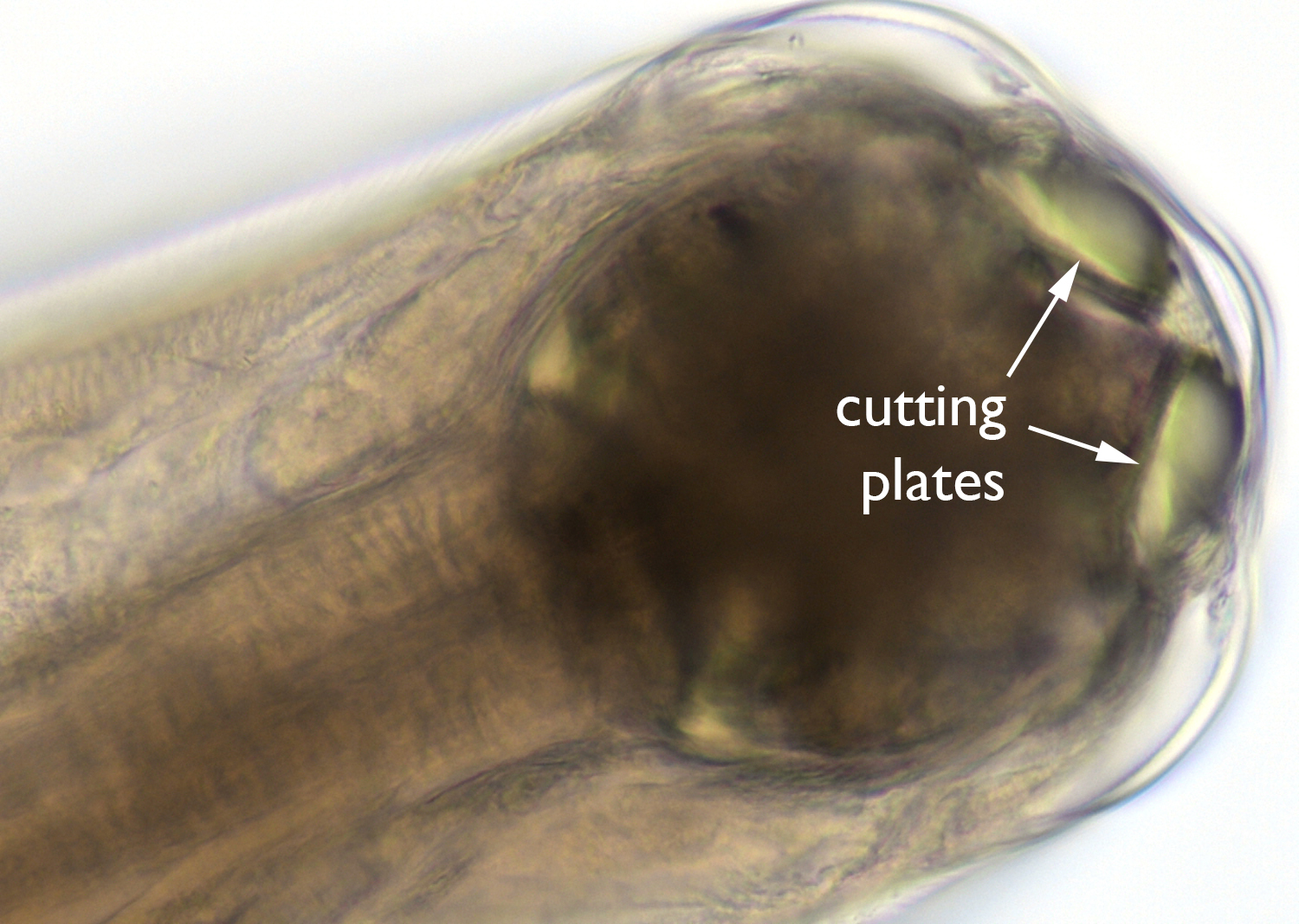This image is a close-up photograph of a unique, cylindrical organism or object, appearing from the lower left corner against a white background. The entity, which might be some form of amoeba, germ, or bacteria, exhibits a cylindrical body and head featuring a transparent, almost translucent surface. The body reveals intricate interior details illuminated by light shining through it. The coloration includes a mixture of beige, dark and light grays, and rusty red tones.

On the top and wrapping around the open end of this cylindrical object—which is situated on the right side—is a reflective white surface, highlighting the structure's clarity. Inside this opening lies a dark brown area, possibly a mouth or an eye, surrounded by what seem to be half-circle, 3D-like objects that could be cutting plates. These green half circles are emphasized by white text within the image, with arrows pointing directly to them and labeling them as "cutting plates." Despite the ambiguity surrounding its exact nature, this translucent cylindrical entity features distinct anatomical components that suggest it might have functional parts like a maw or cutting mechanisms.